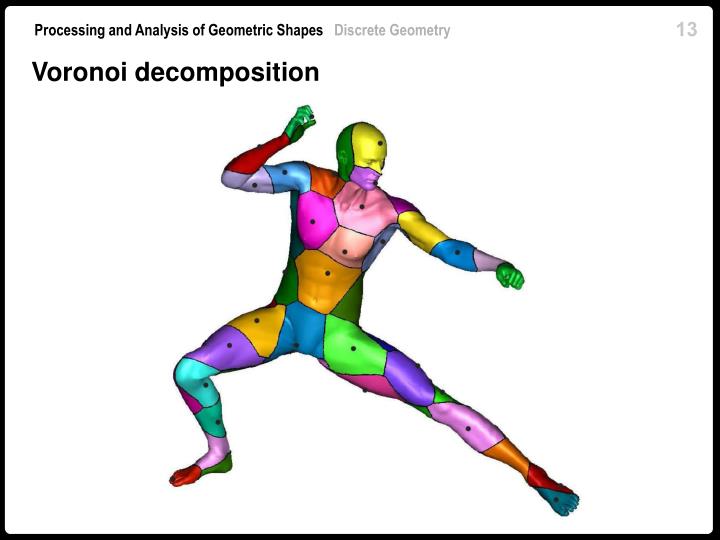This image appears to be a digitally created or book-like page, possibly from a magazine or educational material, surrounded by a black border. At the top of the image, the text prominently reads "Processing and Analysis of Geometric Shapes," with "Discrete Geometry" and "Voronoi Decomposition" written underneath in slightly fainter text. The number 13 is visible in the top right corner.

In the center, there is a colorful 3D model or drawing of a human figure striking a dynamic pose resembling a martial arts stance. The figure's right leg is bent with the foot facing right, while the left leg is extended outward. The right arm is raised, and the left arm stretches out parallel to the extended leg. The body of the figure is divided into approximately 20 to 30 geometric shapes, each marked with a central black dot and colored vividly in hues of pink, yellow, green, blue, red, purple, and other shades. The image conveys a blend of technical and artistic elements, suggesting a study or representation of geometric decomposition applied to human motion.